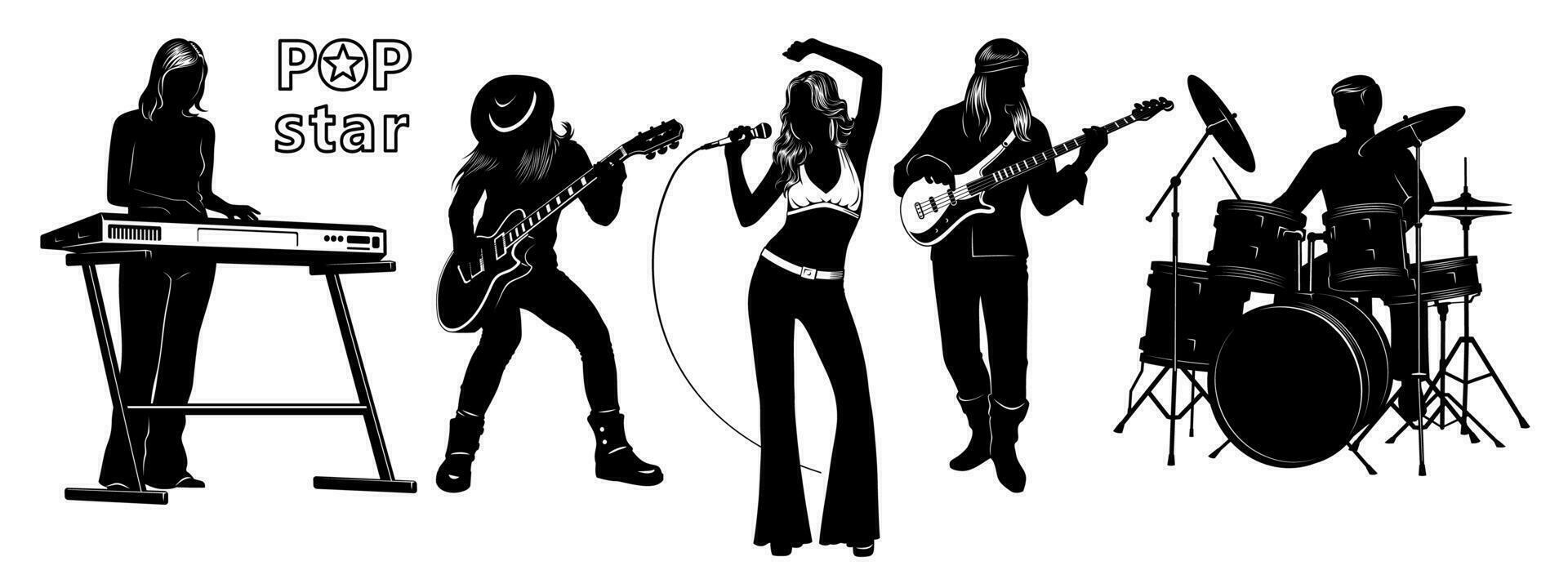This black-and-white image features a silhouetted band against a solid white background, with the text "Pop Star" in the upper left corner, where the O in "pop" has a star in the center. From left to right, the band members are depicted in black outlines: First, a woman stands at a keyboard with tall black legs; moving right, a man with long hair and a cowboy hat plays an electric guitar; the central figure is a singer with long hair wearing a white bikini top and a white belt, holding a microphone in her right hand with her left arm bent behind her head. To her right is another man with long hair playing a white bass guitar standing in a relaxed stance. The scene concludes with a drummer on the far right, surrounded by a detailed drum set with black accents, actively playing. The overall composition highlights the band members and their instruments with a stark, minimalistic flair.